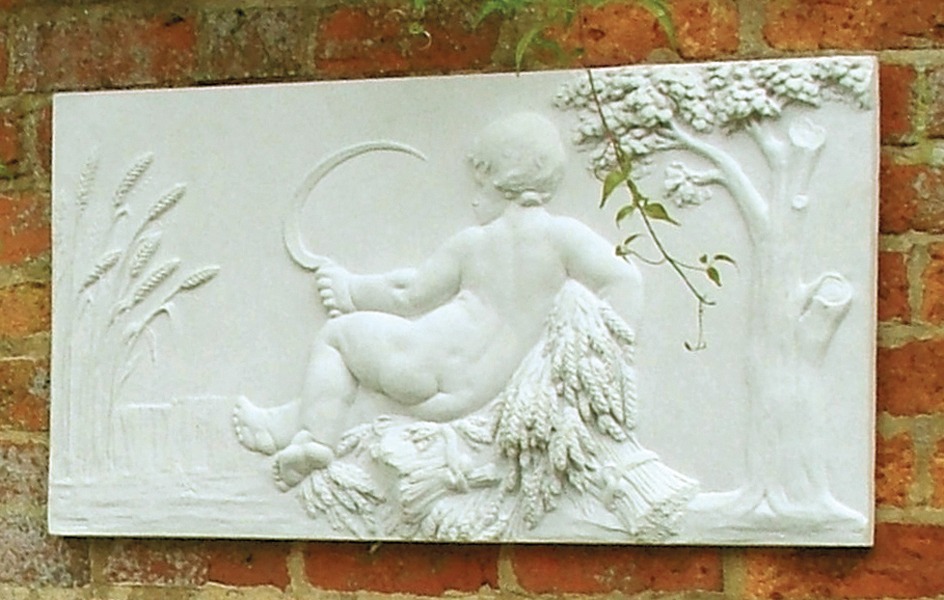This outdoor image features a detailed relief sculpture mounted on an aged, stained red brick wall. The three-dimensional artwork is predominantly white and depicts a cherub-like child in an angelic pose, seated and looking into the distance. The child is completely naked, showcasing his head, back, buttocks, legs, and feet, and he holds a scythe in his left hand. The cherub is reclining on bushels of wheat, with additional sprouting wheat visible on the left side of the piece. On the right side of the sculpture, a tree with leaves is present, and there's a tree branch extending above the relief from a tree beyond the wall. The scene is surrounded by elements of nature, including plants under and around the child, enhancing the serene and pastoral ambiance of the artwork.